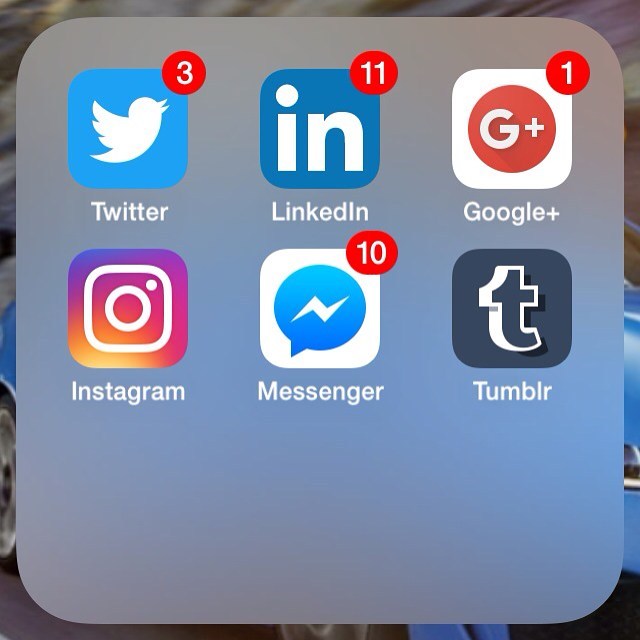A photograph, presumably taken from someone's pocket, showcases the app list on an iPhone screen. The apps are organized in a folder likely intended for communication or social media, containing Twitter (now known as X), LinkedIn, Google Plus, Instagram, Messenger, and Tumblr. The iPhone screen displays several notifications: three for Twitter/X and eleven for LinkedIn, lending a sense of overwhelming digital activity. The screen's background hints at an image capturing a nighttime sky, emitting a slightly fiery glow, though this is not fully evident. The composition suggests an almost romantic aesthetic, adding a layer of visual intrigue.